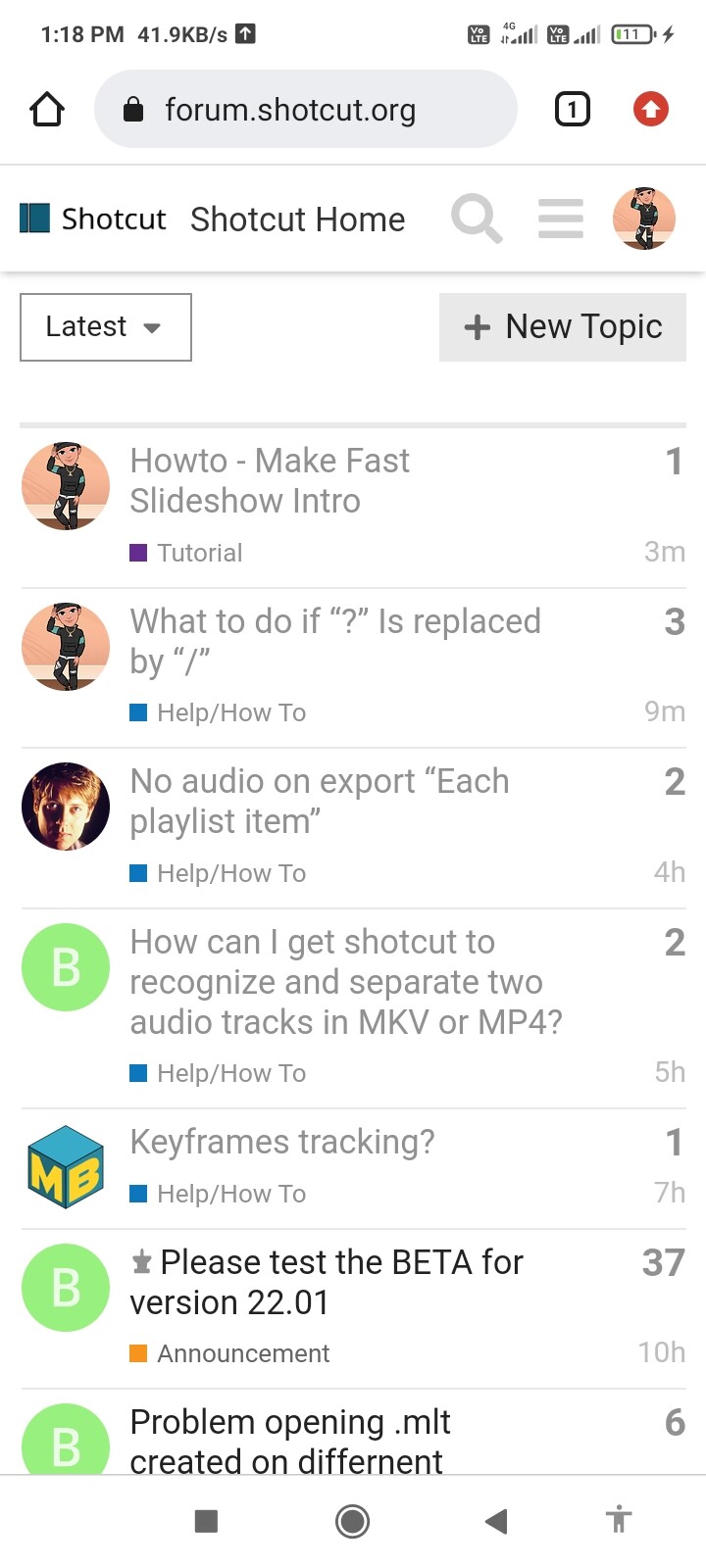The screenshot captures an interface with a white background at 1:18 PM and a battery level at 11% with a charging symbol. At the top, there is a search bar displaying the URL "forum.shortcut.org." Various icons are present including a home icon, a square with the number "1," and a red circle with a white upwards arrow.

Below the search bar, there's the "Shortcut" logo followed by "Shortcut Home." Next to this, you can see a magnifying glass (search icon), a hammer icon, and a profile picture. The screen displays options like "Latest" and a gray rectangle labeled "New Topic."

A series of posts are also visible. The first features a profile picture of a cartoon character and the title "How to make fast slideshow intro" with "1.3M" viewers. This is followed by another post with the same profile picture titled "What to do if question mark is replaced by /" with "3.9M" viewers. 

Further posts include a man’s profile picture with the title "No audio on export" and a viewing time of "2.4H," and another titled "How can I get Shortcut to recognize and separate two audio tracks in MKV or MP4" with "2.5H," represented by a green circle with a white "B." Another post features a blue cube with "M" and "V" in yellow titled "Keyframes Tracking" with "1.7H" views and is marked by the same green circle with the white "B."